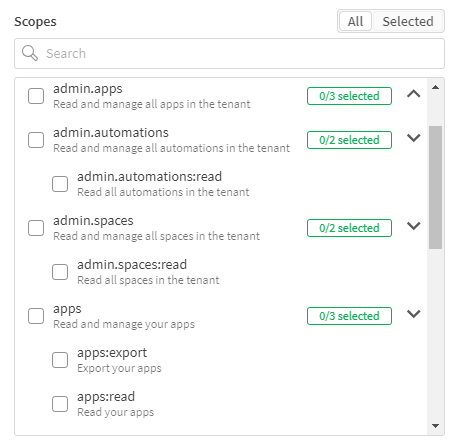A screenshot featuring a user interface with a clean white background and dark gray text. Dominating the upper left corner is the heading "Scopes." To its right, a toggle button allows users to switch between "All" or "Selected." Just beneath, a search bar offers quick navigation. Four green rectangles, each containing the word "Selected" and a corresponding number, align vertically along the right side of the screen.

The central section of the screenshot presents a list of options, each accompanied by an empty square checkbox. The options are listed as follows:
- Admin.Apps
- Admin.Automations
- Admin.Automations: Read
- Admin.Spaces
- Admin.Spaces: Read
- Apps
- Apps: Export
- Apps: Read

On the far right, a vertical slider bar facilitates easy navigation through the page.